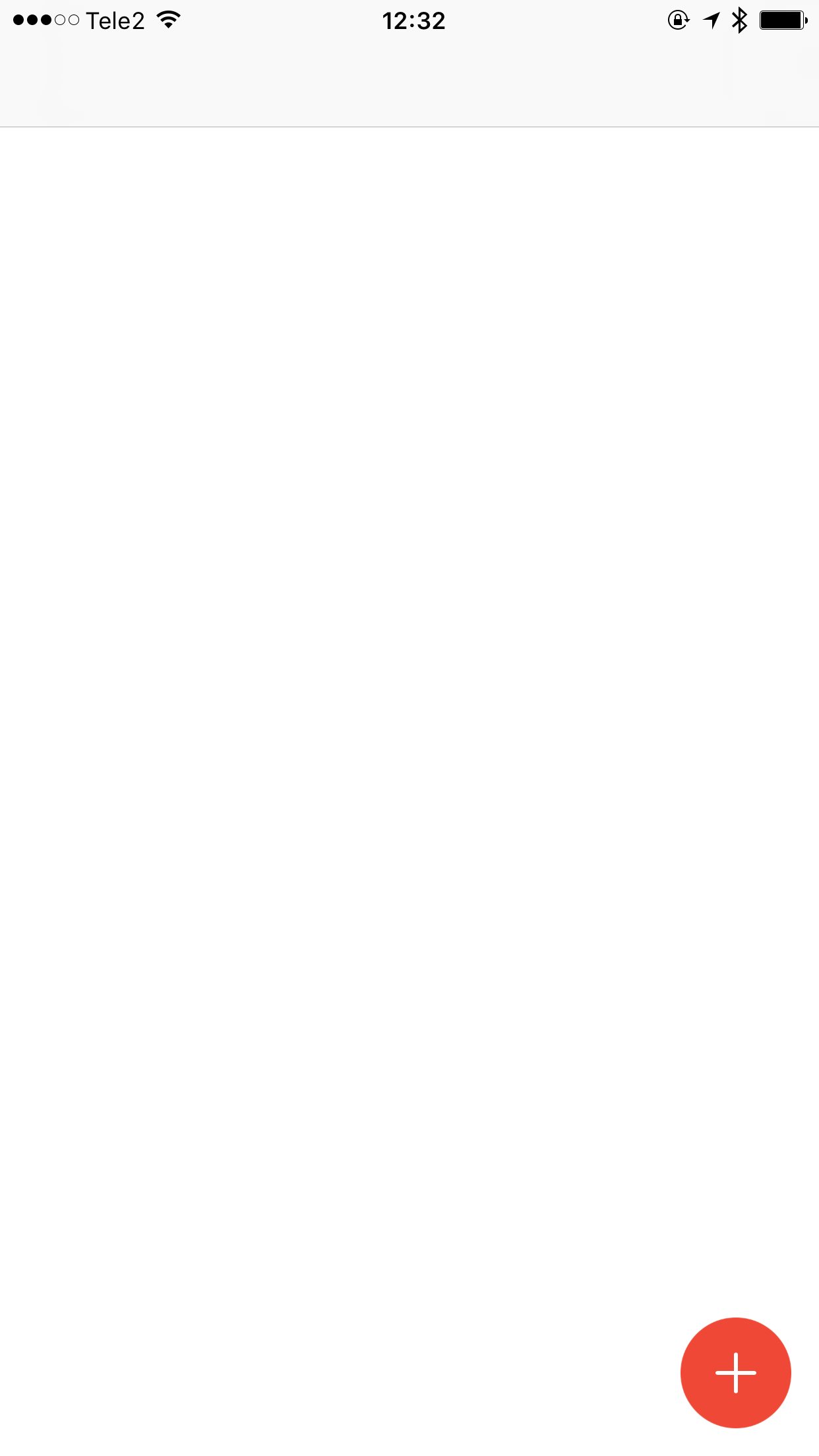Screenshot from a mobile device with a predominantly white background. The top section of the screen displays the status bar including three out of five signal bars for the carrier "TELE2." The time shown is 12:32. Various icons are present: a lock icon, a black location arrow, a Bluetooth icon, and a nearly full battery icon. A gray line runs horizontally across the top. The bottom of the screen features a single element: a prominent red circular button with a plus sign. The rest of the screen is entirely white and devoid of any additional content.